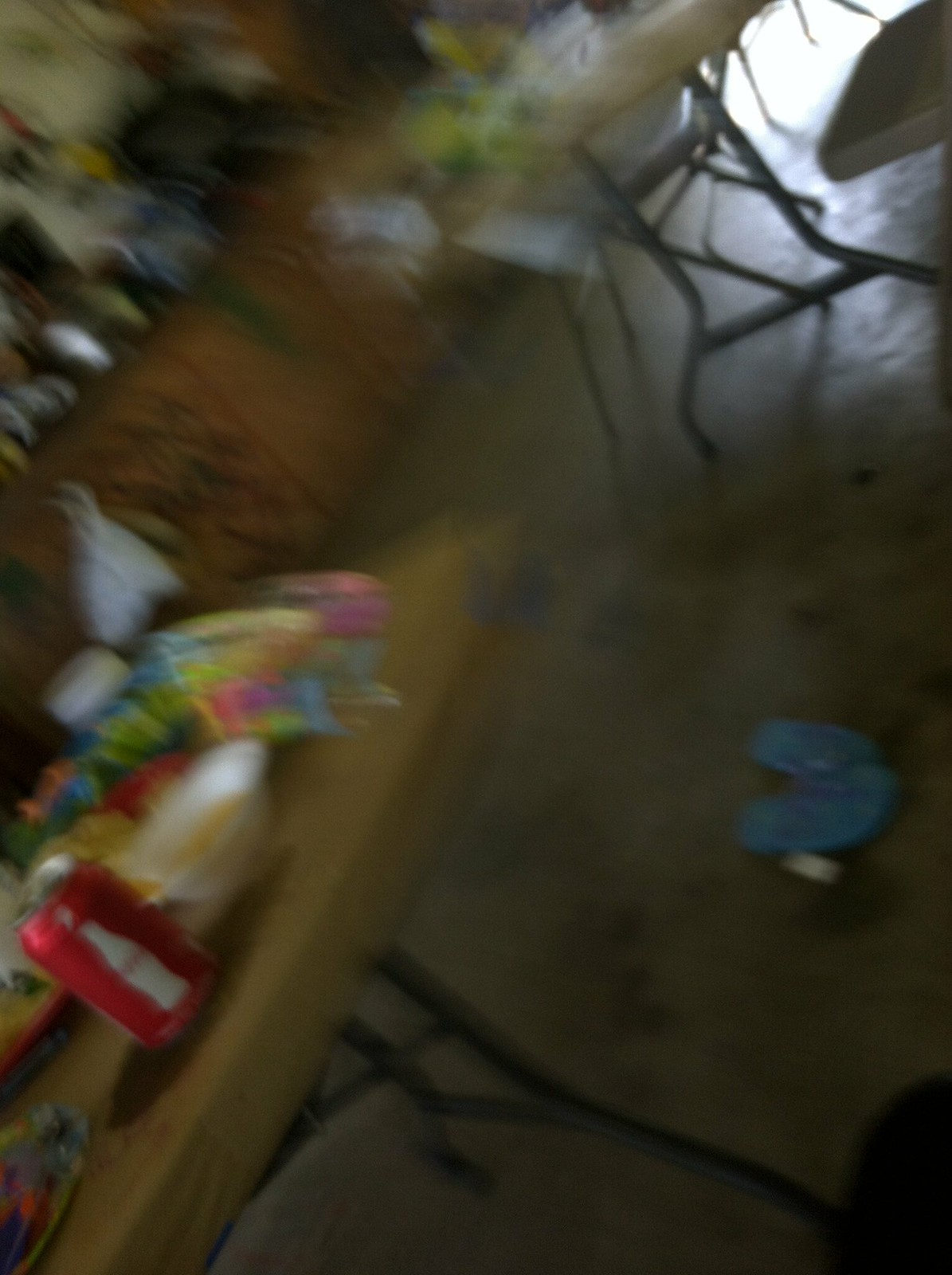The blurry photograph appears to be taken in a garage or a kitchen setting, featuring a gray concrete floor and wooden cupboards in the background. Central to the image are two folding tables with black stands and light brown tabletops, seemingly set up for a party. The table to the left is cluttered with various items, including an open can of Coke, a small white foam bowl, and several brightly colored objects potentially linked to party supplies like balloons or candy. Blue flip-flops are noticeable on the floor near a white object. Folded chairs are arranged around the tables, and cabinets with assorted items, possibly tools or plastic containers, are visible in the backdrop. The right-hand side of the image features a bright, reflective area suggesting sunlight streaming in, likely from a garage door. Despite the overall blurriness and muted colors, the scene hints at a casual, possibly child-oriented celebration.